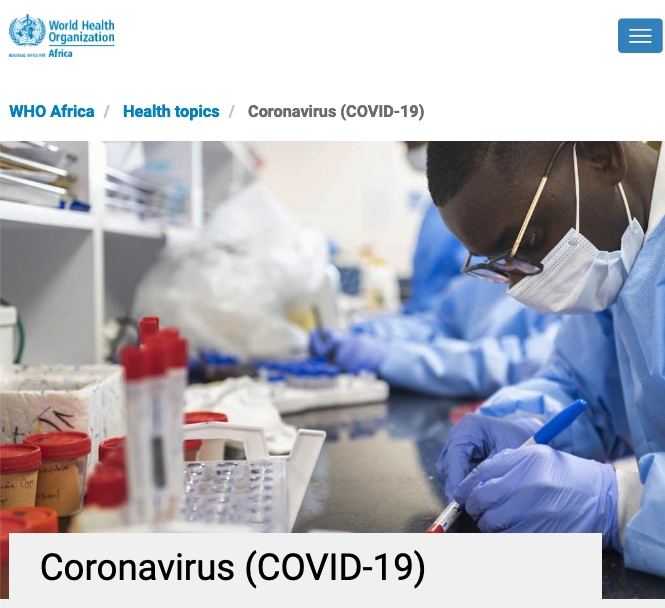The image depicts the official website of the World Health Organization (WHO), specifically the Africa regional section. In the top left corner, there is a distinguished blue symbol, representative of WHO. Adjacent to the symbol, "World Health Organization" is prominently displayed. Directly underneath this title, the word "Africa" can be seen, indicating the regional focus of the webpage.

In the upper right corner of the screen, a blue square icon with three vertical lines is visible, which likely serves as a menu button for navigation. The main content area features a photograph prominently centered. Above the photograph, a navigation breadcrumb trail directs users through sections of the website, starting with “WHO Africa” in blue text, followed by a slash, “Health Topics” also in blue, another slash, and then "Coronavirus" in gray with "COVID-19" enclosed in brackets.

The central photograph portrays a laboratory scene. A scientist or doctor is seen standing at a tall countertop, holding a blue marker and carefully writing on the side of a blood tube. In front of them, a flat container with multiple holes for holding tubes is visible. Another person, also dressed in a blue lab coat, white surgical mask, and blue gloves, stands behind the primary subject, engaged in a similar task. This detailed depiction highlights the scientific efforts and meticulous procedures involved in the ongoing research and management of the COVID-19 pandemic.